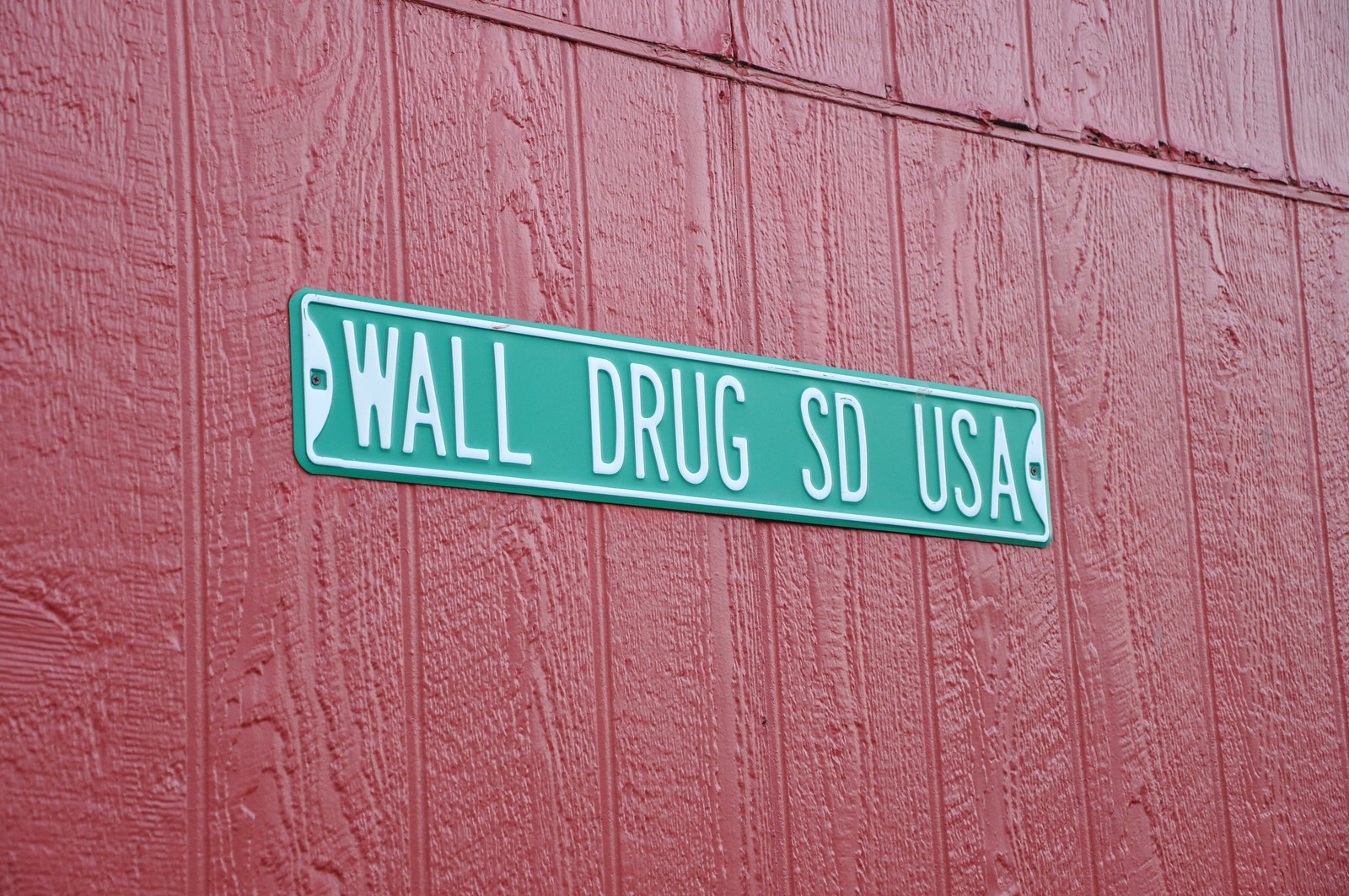The image appears to be taken outside, showcasing the façade of a rustic barn with vertically aligned wooden planks, painted in a vibrant red. The wood grains, running parallel to the planks, are clearly visible, adding a textural element to the scene. Centrally mounted on this red wooden wall is a long rectangular sign with a green background and a distinct white border. On either end of the sign, there are small square holes for mounting. The sign itself features bold, all-capital white letters, spelling out "WALL RUG S-D-U-S-A." The simplicity of the composition, with nothing else in the frame, emphasizes the sign and the texture of the weathered barn wall.